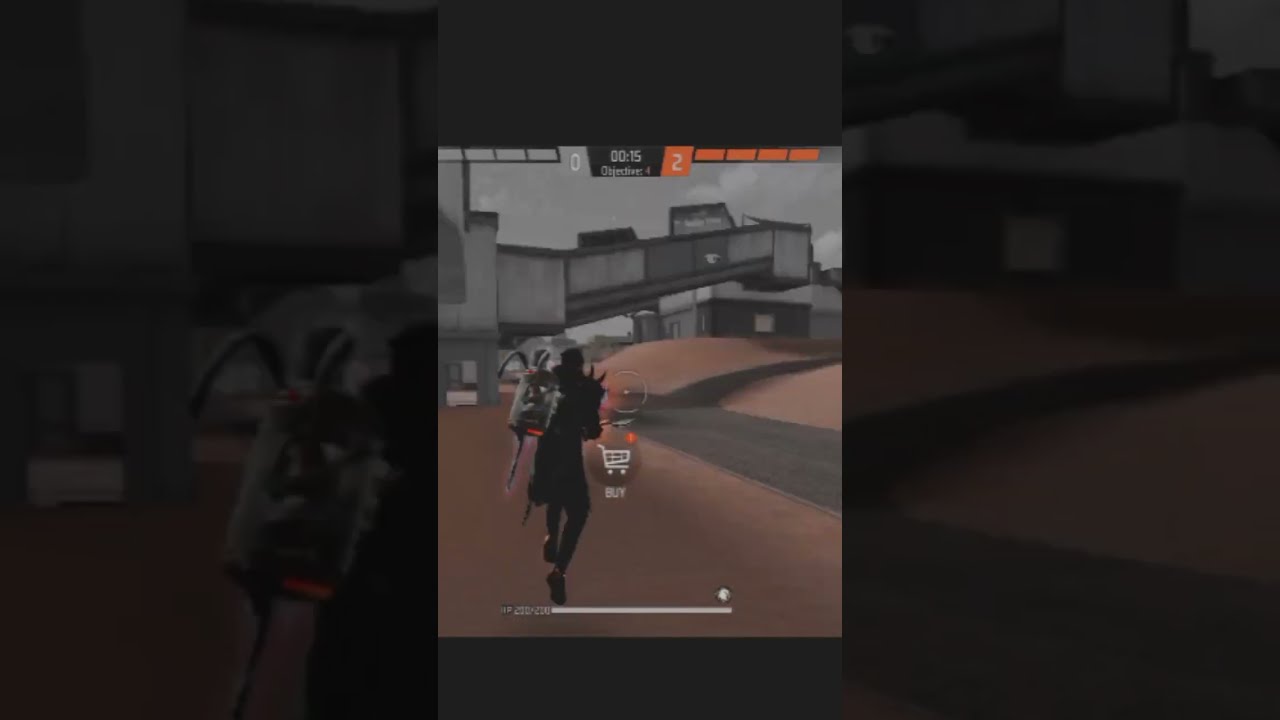In the midst of a completely black background, there's a clear and brighter square image that seems to depict a scene from a video or mobile game. In the center of this image stands the black silhouette of a person, likely a soldier, with a backpack on their back. To the right of this figure is a small shopping cart icon labeled "buy," suggesting the option to purchase items within the game. The ground beneath them is brown, interspersed with patches of red, and there's a paved roadway running horizontally through the middle of the screen. A thin white bar at the bottom may indicate time elapsing. Above this scene, a structure that appears to be a tunnel or a covered bridge can be seen, with additional buildings and cloudy gray skies in the far background. At the top of the image, the text "objective four" is displayed alongside a timer showing '00:15'. An orange number '2' and a gray '0' are also present, possibly indicating the game's score. The surrounding black background to the left and right of the central image is darker and less detailed, with vague outlines barely visible.